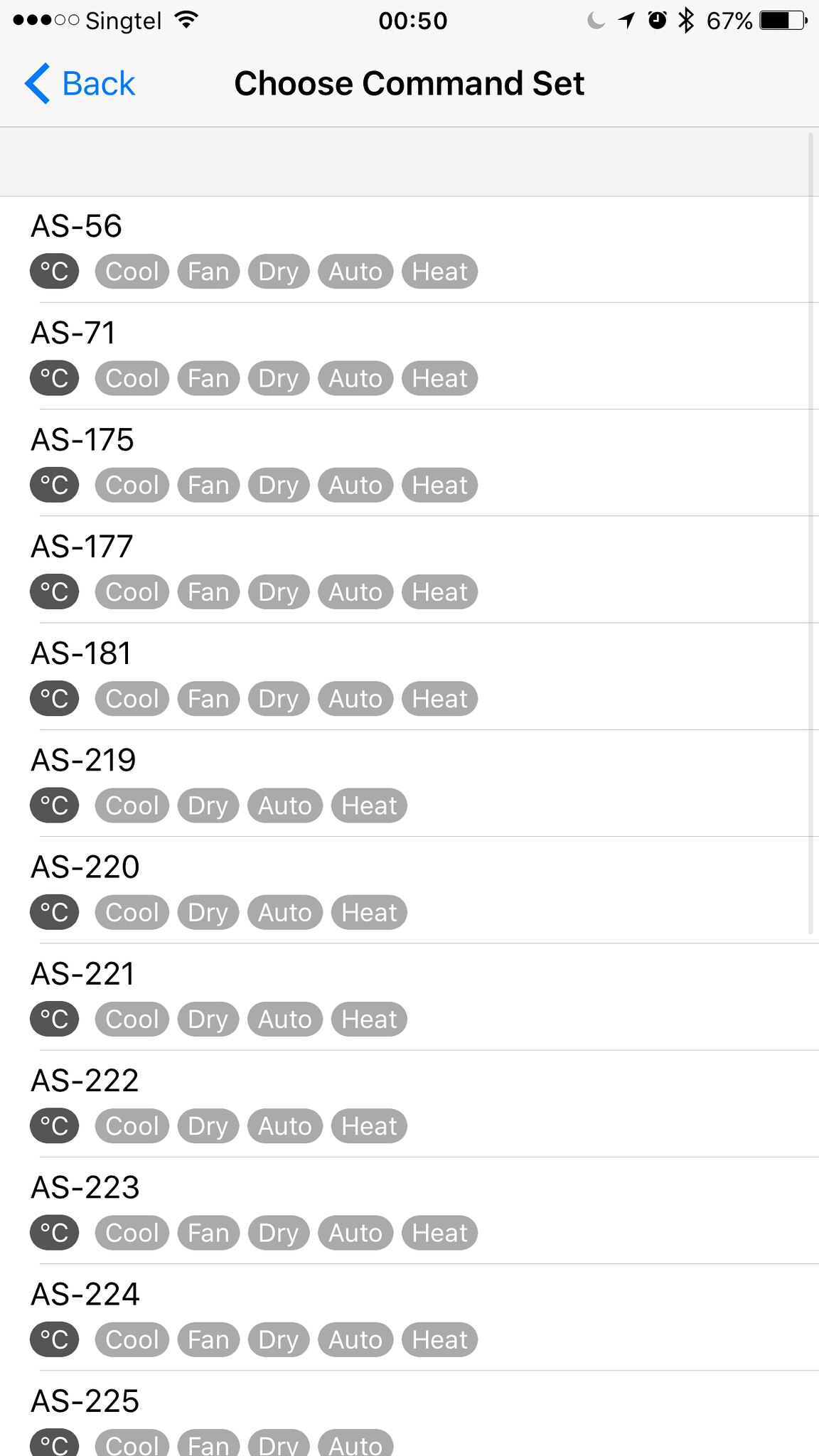A smartphone screen displaying a dryer control app is depicted in the image. At the top left corner, five signal strength indicators are visible: three filled black dots and two empty ones, with "Singtel" (short for Singapore Telephone) and a Wi-Fi symbol next to them. The center of the status bar reads "00:50," possibly indicating a timer set to 50 minutes, and the right side shows several icons, including a recognizable Bluetooth symbol and a battery icon displaying 67% charge.

Below the status bar, the top section of the app interface reads "Choose Command Set." To its left, "Back" is written in blue text, accompanied by a blue left-pointing arrow suggesting a return to the previous menu. The main content area consists of twelve lines of commands likely pertaining to different dryer models. Each line begins with a model number, such as "AS-56," "AS-71," "AS-175," continuing with models like "221," "222," "223," "224," and "225."

Each model number is followed by a dark oval displaying temperature in degrees Celsius. Adjacent to these are lighter grey ovals with white text offering various settings: "cool," "fan," "dry," "auto," and "heat." Notably, models starting with "200" initially lack the "fan" option, listing only "cool," "dry," "auto," and "heat." However, the "fan" option reappears for models 223 and higher, returning to the sequence "cool," "fan," "dry," "auto," and "heat."

The interface provides a comprehensive view of the command options available for controlling different dryer models, indicating a sophisticated application designed to cater to varied user requirements.